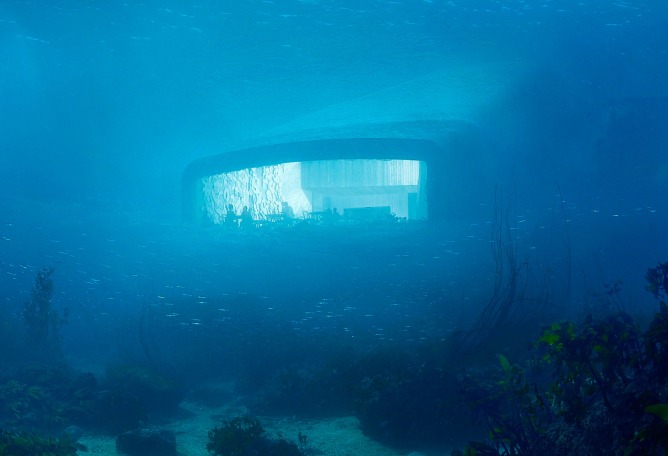The image depicts an underwater scene, showcasing a submerged vehicle resting on the ocean floor. The water appears murky, with a noticeable greenish-yellow tint near the bottom. Surrounding the vehicle are various aquatic plants, resembling underwater trees and bushes, which display shades of green and yellow. Small bubbles rise from the seabed, ascending through the water. The vehicle, partially illuminated from within, emits a faint, glowing light, adding an aura of mystery to the scene. The overall backdrop of the image is dominated by the deep blue hues of the surrounding water, enhancing the sense of depth and immersion in this underwater world.